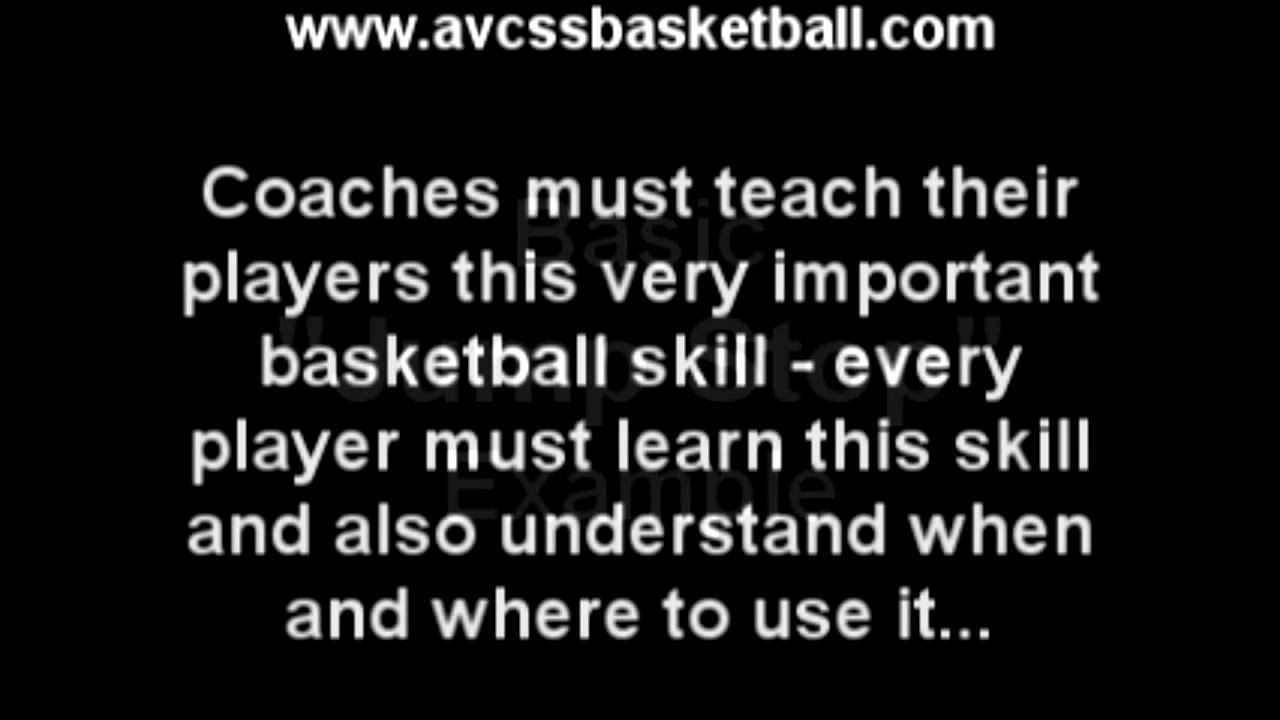The image features white text on a solid black background. At the top, in smaller white letters, it reads "www.avcssbasketball.com." Below this URL, in a larger white font, the message states: "Coaches must teach their players this very important basketball skill. Every player must learn this skill and also understand when and where to use it..." The text is center-aligned, and the first letter "C" in "Coaches" is capitalized while the rest of the text is in lowercase. Additionally, faint words can be seen in the background, including "basic" and "example." The overall composition gives the impression of a teaser or an instructional slide, likely related to basketball coaching strategies.